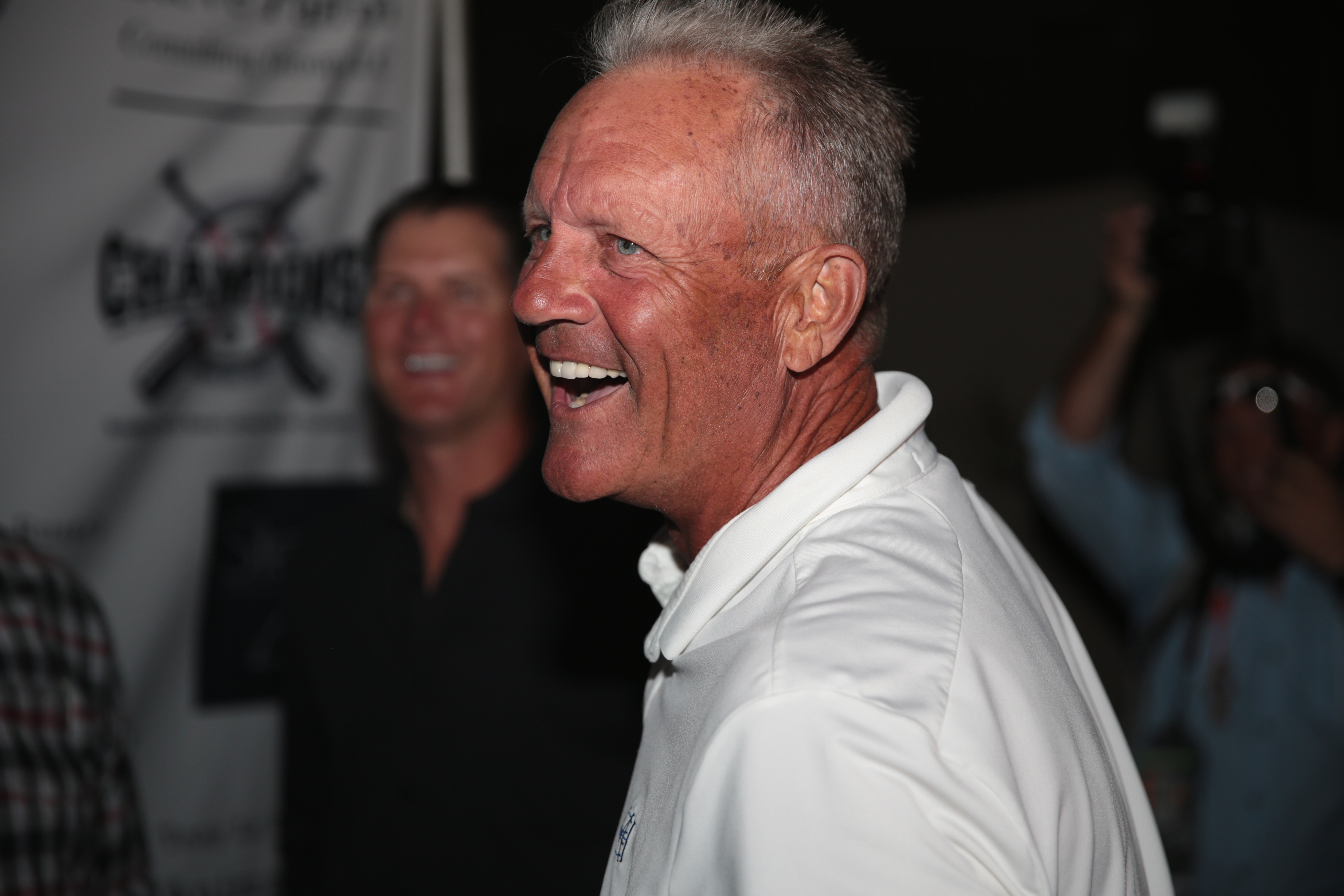In this image, we see legendary third baseman George Brett, celebrated for his time with the Kansas City Royals. He is captured standing sideways, oriented towards the left of the photo, but his head is turned slightly to face the camera with a broad smile, showing his white teeth and revealing his pale blue eyes and short, graying hair. Brett is wearing a white collared shirt and appears to be at some sort of evening or nighttime event possibly honoring him, surrounded by an atmosphere of celebration. In the blurry background, various people are visible: a man with rosy cheeks in a black shirt, another in a black and red plaid shirt, and someone holding a camera. There is also a large white poster with crossed baseball bats and the repeated text "champions," hinting at Brett's honored status in the baseball world. The background overall has a festive feel, with numerous smiling faces contributing to the sense of celebration.